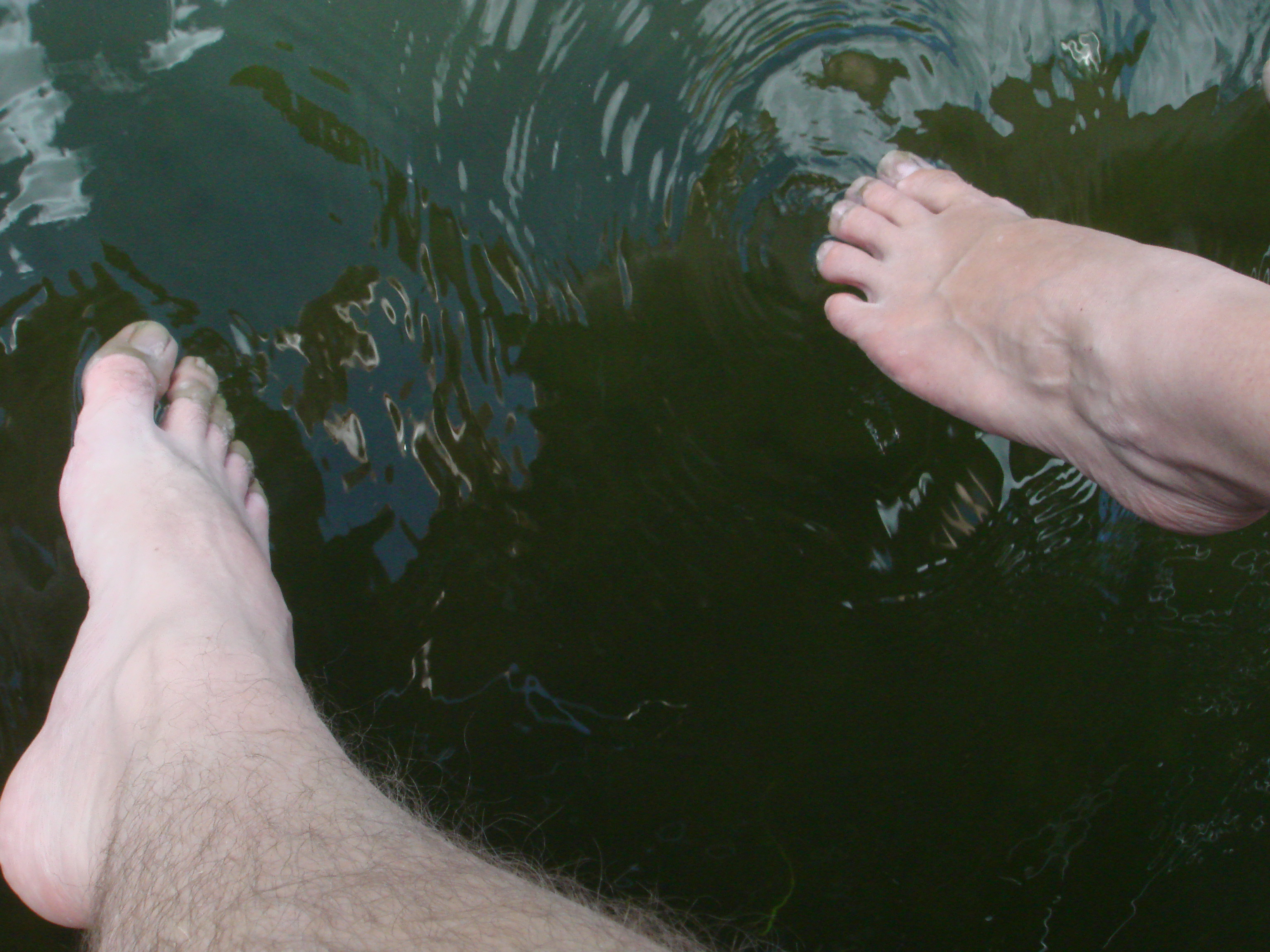The image captures an intimate moment of two individuals dipping their feet into a dark, murky body of water with a green tint, likely a lake or river. The foot in the lower left corner of the frame belongs to a person with a larger, hairy leg that extends up to the calf, speckled with sand on their toes. Positioned towards the upper right corner is a slender female foot, visibly veined with thin skin and also adorned with sandy toes. Both feet are pointed slightly downward into the water, creating gentle ripples on the surface. The background is predominantly the murky, bluish-green water, contributing to the natural and serene setting from a bird's-eye view.